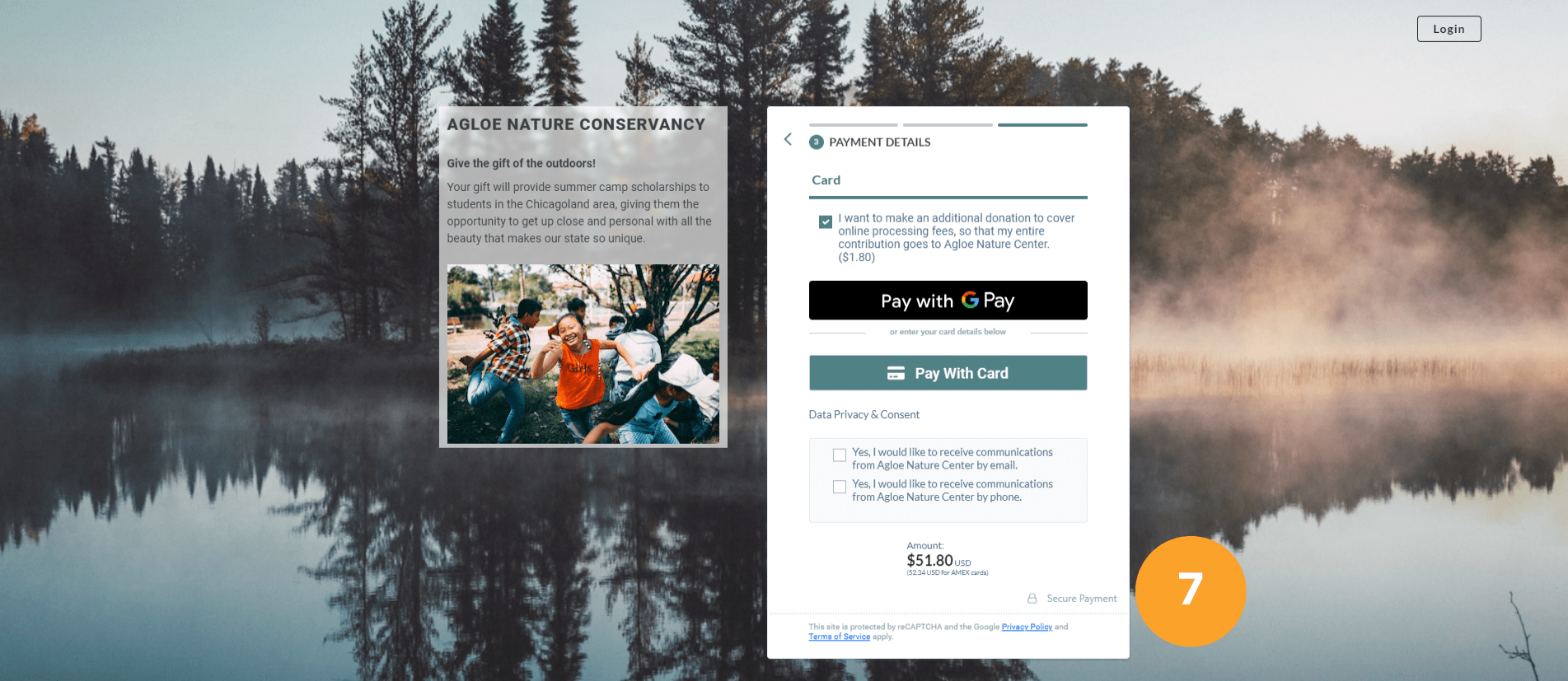Screenshot of the Awago Nature Conservatory Donation Page

This image is a screenshot of the donation page for the Awago Nature Conservatory. The background of the page features a serene early morning scene of a pond or lake shrouded in mist, with the soft light of dawn just beginning to break through. The tranquil water beautifully reflects the surrounding trees, adding to the picturesque quality of the scenery.

In the top right-hand corner of the screenshot, there is a "Log In" option. Below it, a gray rectangle contains a poignant appeal for donations: "Awago Nature Conservatory - Give the Gift of Outdoors." The text explains that contributions will provide summer camp scholarships to students in the Chicagoland area, offering them the chance to experience the unique natural beauty of the state up close.

At the center of the screen, a larger white rectangle serves as the main donation form. Here, users are prompted to enter their payment details, including their card number. There is also an option selected for making an additional donation of $1.80 to cover online processing fees, ensuring that the entire contribution amount of $51.80 USD goes to the Awago Nature Conservatory.

Payment methods available include "Pay with Google Pay" and "Pay with card." Beneath the payment options, there is a section labeled "Data Privacy and Consent," where users can manage their consent preferences. Notably, the bottom right-hand side of this payment window features a small circle with the number 7 inside.